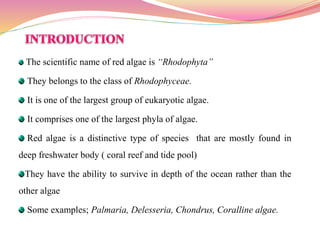The image appears to be an informational slide, resembling those found in a textbook or academic project. It features a border with pinkish and yellowish waves at the top. Below this border, in pink text on the left-hand side, the word "Introduction" is prominently displayed. Each line of information is marked with a green bullet point. The content begins with the scientific name of red algae, "Rhodophyta," which is italicized. The subsequent bullet points explain that Rhodophyta belong to the class Rhodophycae and are one of the largest groups of eukaryotic algae. It is further noted that red algae comprise one of the largest phyla of algae. Red algae are distinctive species mostly found in deep freshwater bodies, coral reefs, and tide pools, and they can survive at greater ocean depths compared to other algae. The slide also provides examples of red algae species, such as Palmaria, Delesseria, and Chondrus.